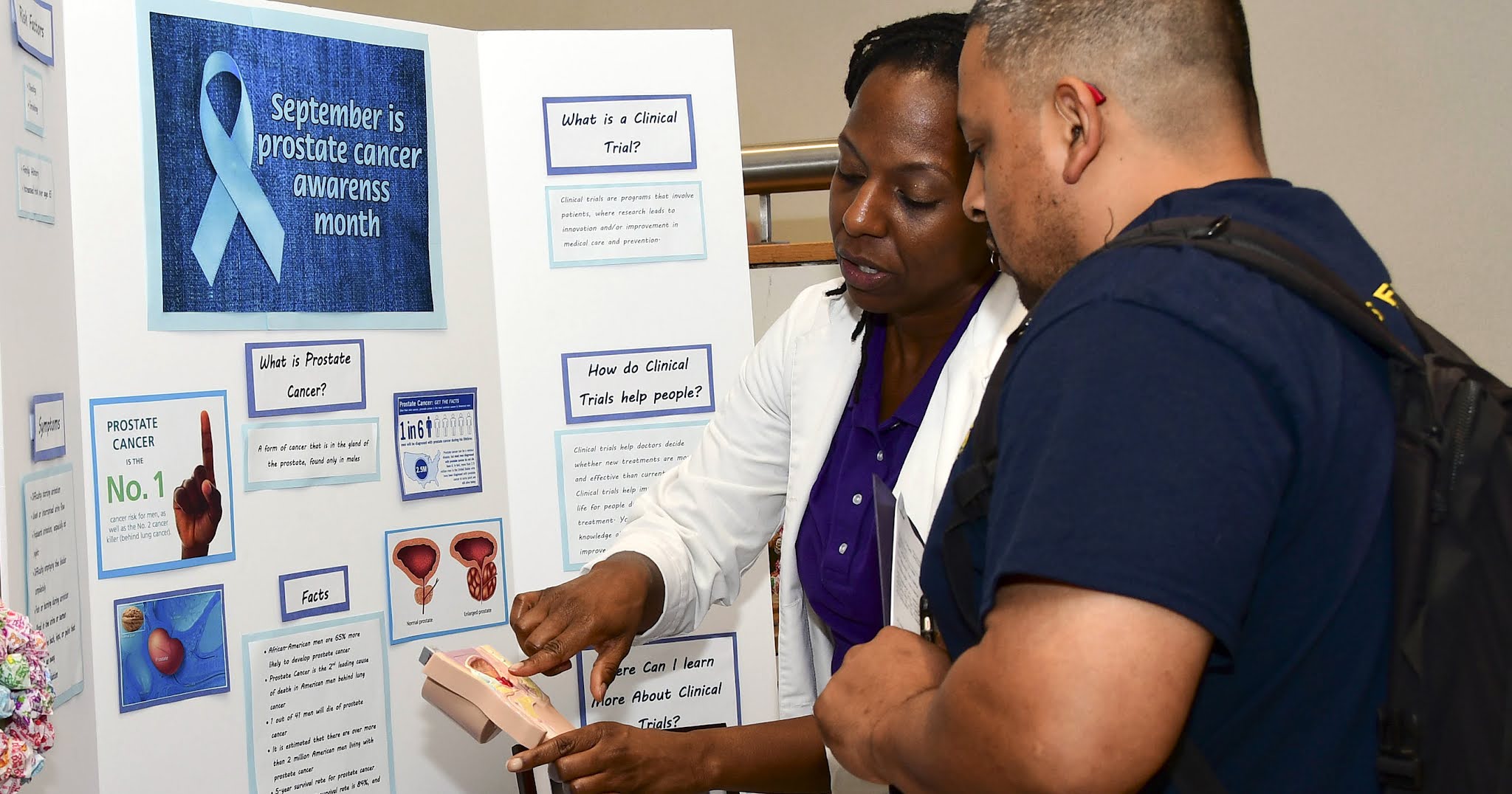In this image, a black woman with black hair, dressed in a white doctor's coat and a blue polo shirt, is standing beside a Mexican man who has gray and black shaved hair, is wearing a blue t-shirt, and is carrying a black backpack. They are standing in front of a large trifold informational medical board, which prominently features a sign at the top reading "September is Prostate Cancer Awareness Month" in blue text, accompanied by a blue ribbon on the left-hand side. The woman, likely a healthcare professional, is holding and pointing at a plastic medical model as she explains something to the man. The board contains several sections with text outlined in blue, including headings like "What is a clinical trial?", "How do clinical trials help people?", and various factual information about prostate cancer. The image is oriented horizontally, similar to a science fair display, with detailed informational snippets designed to educate viewers about prostate cancer.